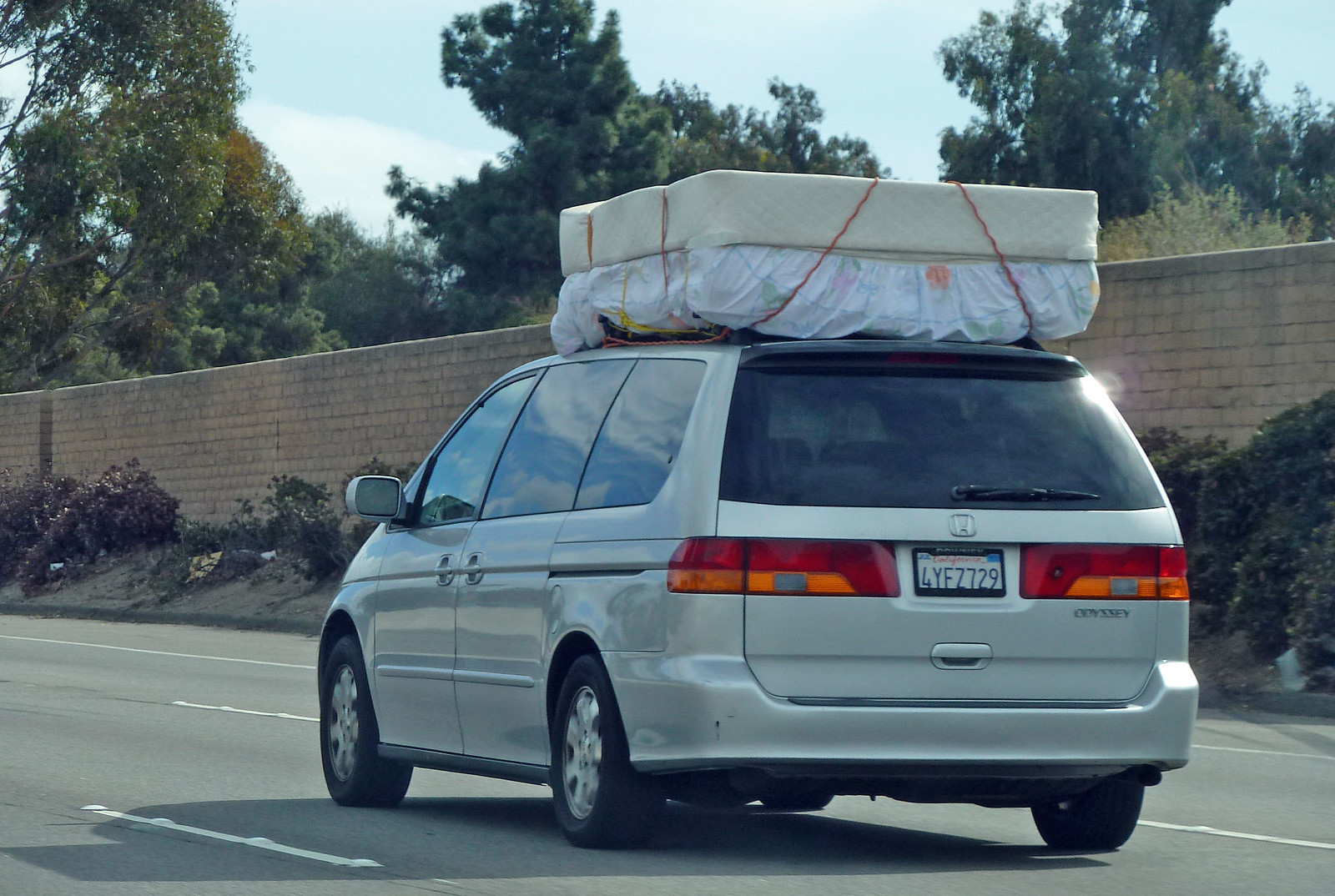In this detailed photograph taken on a freeway, a silver Honda Odyssey minivan with tinted windows and a California license plate 4YFZ729 is prominently displayed in the foreground. The minivan, which is stationary, has two mattresses securely tied to its roof with ropes, suggesting that it might be used for moving. The vehicle features red and orange tail lights, white reverse lights, silver wheels, and a rear door that opens upwards, complete with a windshield wiper. The highway itself consists of three lanes, and alongside the road to the right, there's a sound barrier wall. Behind this wall, tall trees stretch into the clear blue sky with some occasional clouds. Adjacent to the wall, there is a section of earth populated with bushes, adding a touch of greenery to the scene. This detailed and vivid snapshot captures a moment of stillness amidst the bustling activity of the freeway environment.